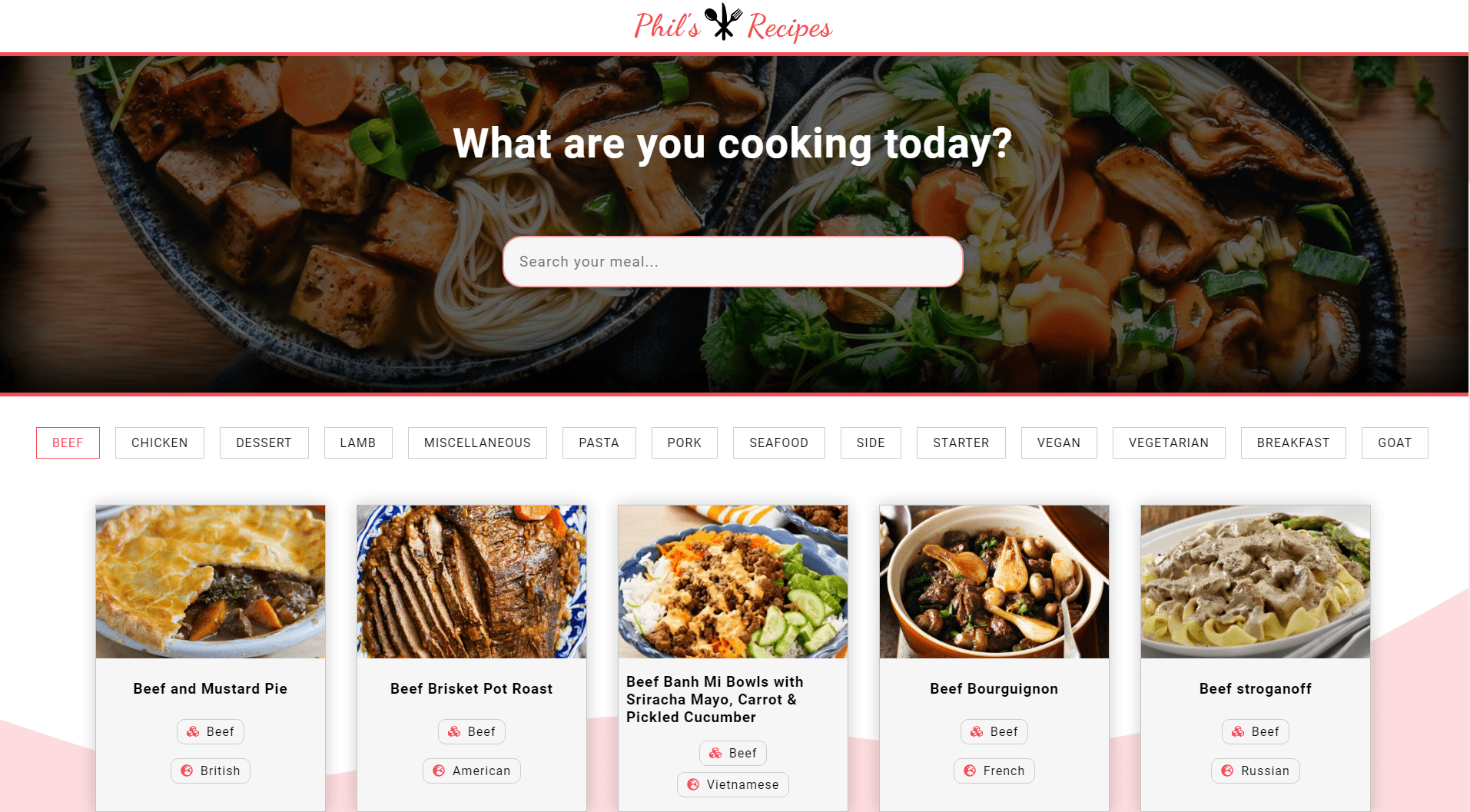The screenshot depicts a vibrant and organized interface titled "Phil's Recipes." At the top of the screen, three crossed kitchen utensils – a knife, spatula, and spoon – serve as the logo. Prominently displayed is the question "What are you cooking today?" in a large white font. Directly beneath this header lies a long, oval-shaped search bar.

The background features two faintly visible dishes, likely vegetarian, showcasing mushrooms, tofu, and noodles. Below the search area, there are various selectable categories including: Beef, Chicken, Dessert, Lamb, Miscellaneous, Pasta, Pork, Seafood, Side, Starter, Vegan, Vegetarian, Breakfast, and Goat.

Farther down, the interface displays five tempting food images. The first image is labeled "Beef and Mustard Pie," accompanied by category buttons for "Beef" and "British." Other visible dish titles include Beef Brisket, Pot Roast, Bánh Mì Bowls, Bò Ngon, and Beef Stroganoff. Each dish is designed to entice the viewer with its visually appealing presentation and easy-to-navigate buttons for further exploration.